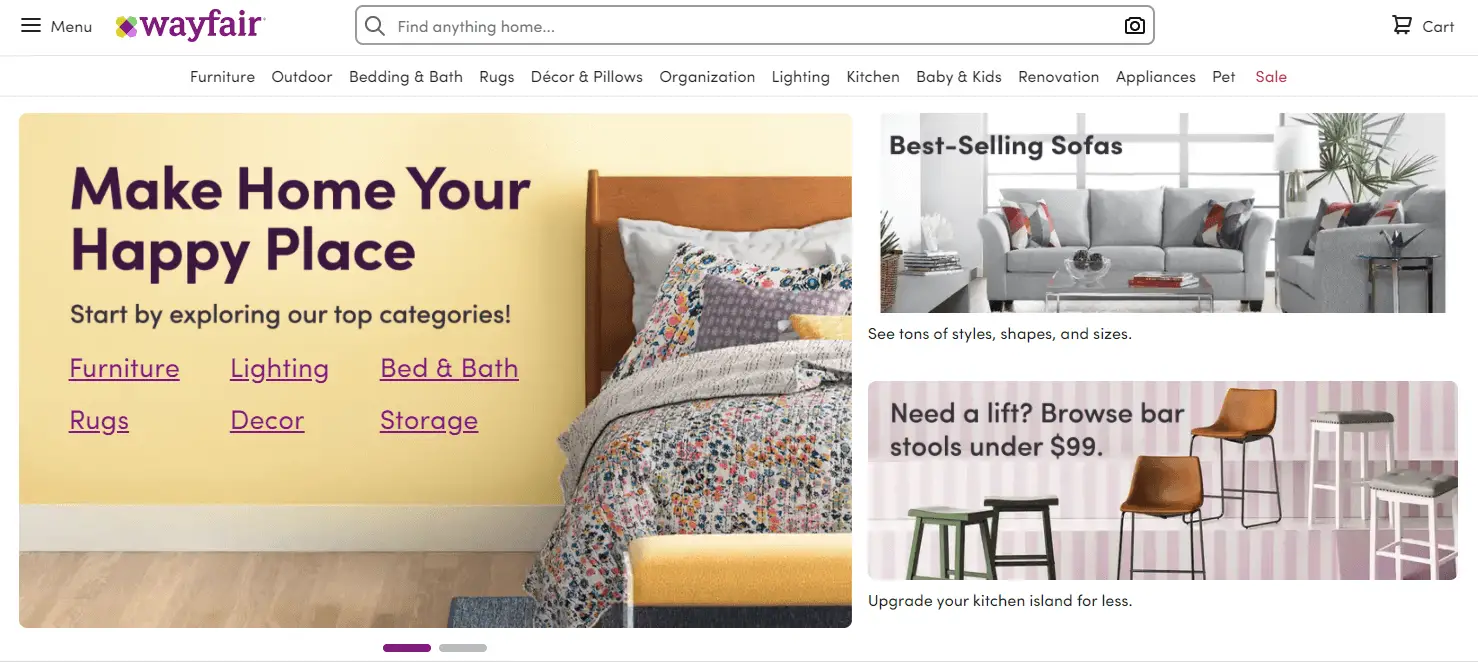This image features the homepage of Wayfair, an online furniture retailer known for its wide range of home decor items. Prominently displayed on the page is the Wayfair logo in a vibrant pink or purple text. The homepage's banner reads "Make Your Home a Happy Place," inviting visitors to explore various categories such as furniture, best-selling sofas, and budget-friendly options like bar stools available for under $99. The overall design is bright and welcoming, geared toward inspiring potential buyers with stylish and affordable home solutions. Despite its appeal, the narrator mentions finding Wayfair somewhat expensive and primarily uses the site for inspiration.